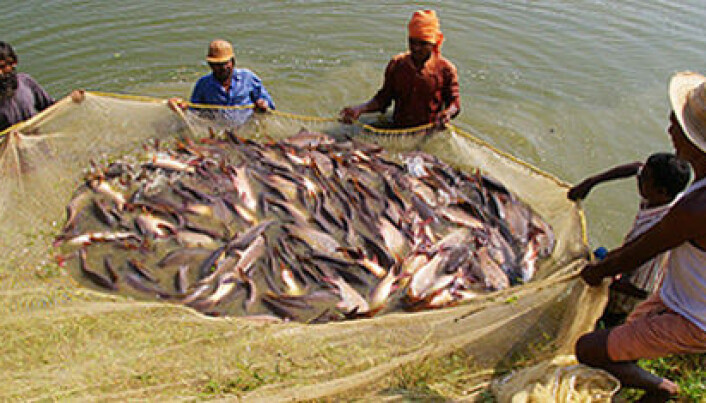In this vibrant and detailed scene, a group of five fishermen, composed of four adult men and one child, are engaged in hauling in their abundant catch of fish with a gigantic net. The group, located waist-deep in muddy, shallow water near the shoreline, works together as they hold different sides of a yellow-trimmed fishing net teeming with fish. The men, who have black skin, are dressed in light, warm-weather clothing, suggesting a tropical climate. One man sports an orange bandana and matching shirt, another wears a blue shirt paired with a tan hat, a third has a gray shirt with a black hat, while the fourth is clad in a white shirt, orange shorts, and a white hat. Diverse headgear, from a wicker hat to a turban wrap, is also notable among the group. The fish, displaying brown tops and white undersides with splashes of red, glisten in the net as the fishermen pull it toward their boat, under a sunny sky. The scene is enhanced further by the visible grass at the bottom edge of the photograph, highlighting their proximity to the shore.